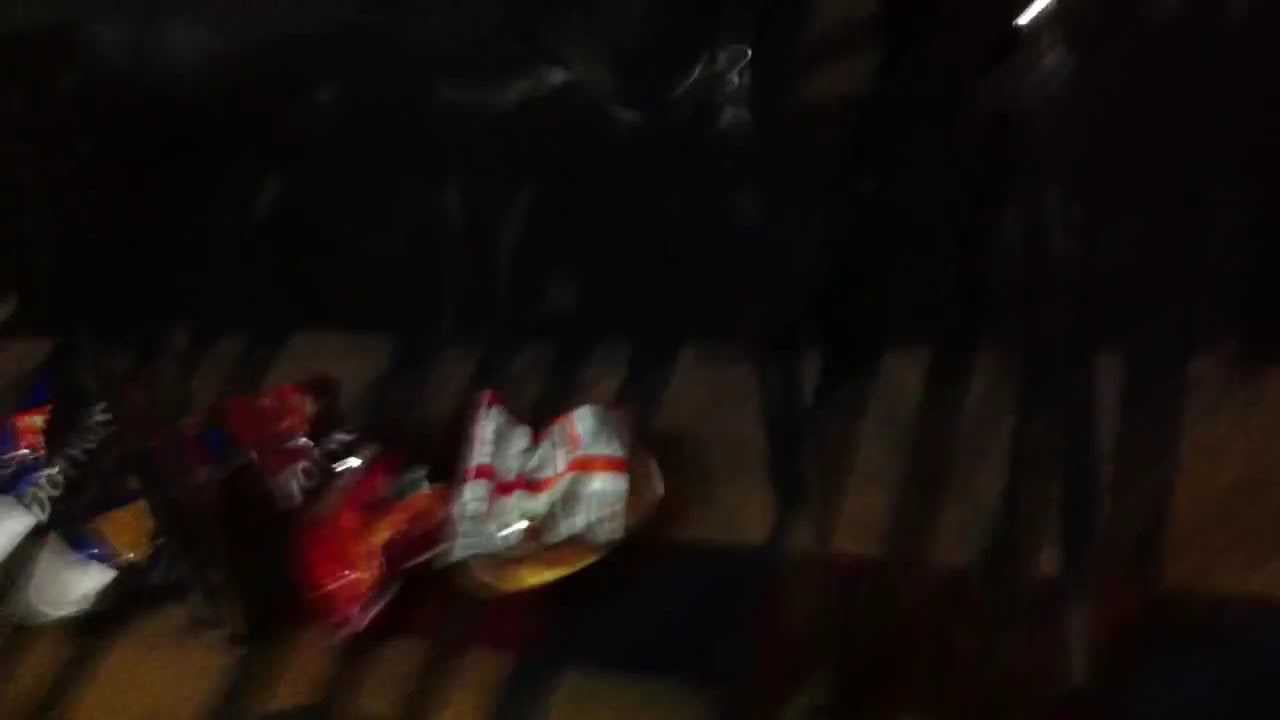This image is a very blurry and poorly lit photo, with an overall dark ambiance except for a dim, amber-hued glow, reminiscent of streetlighting, casting over some items. The lower half of the image appears to have a gray, cement-like surface with this amber glow. What might be shadows or dark strips hang down across the scene, creating a lattice-like effect. On the left side of the image, atop what looks like a table, are three crumpled bags of chips. The first bag, on the far left, is identifiable as a Cool Ranch Doritos bag. Next to it is a classic Nacho Cheese Doritos bag. The third bag, positioned with its backside facing up, reveals only a white base with a red stripe, making its exact contents indiscernible.